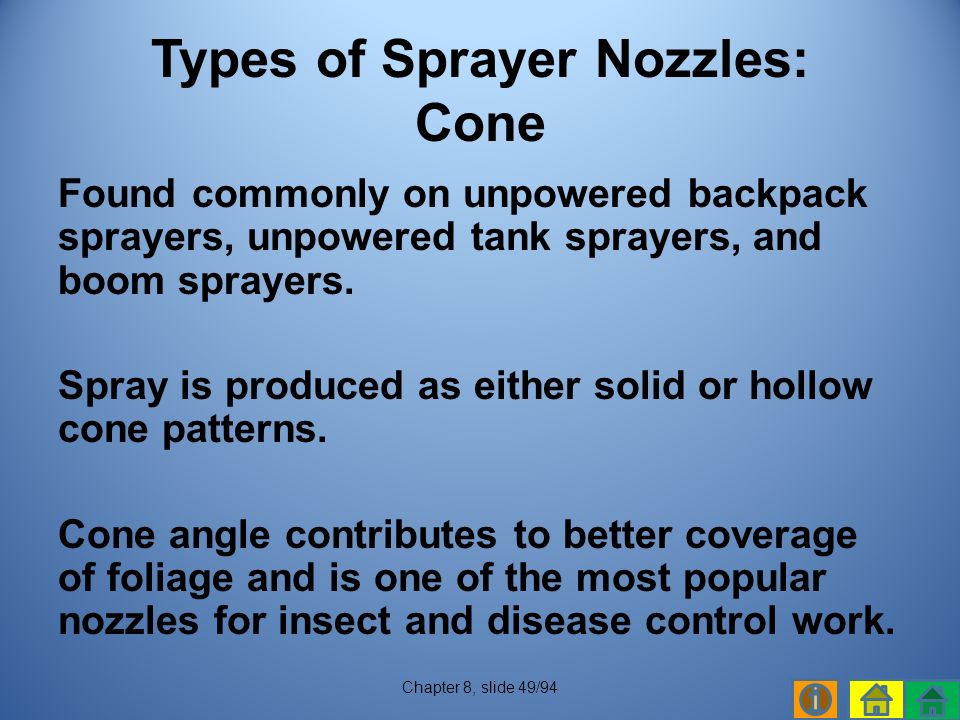The image is a rectangular slide from a presentation or instructional material, titled "Types of Sprayer Nozzles." The background is a rich dark blue color. The text, which is centered and occupies most of the slide, explains the usage and characteristics of cone sprayer nozzles. It states that these nozzles are commonly found on unpowered backpack sprayers, unpowered tank sprayers, and boom sprayers, and notes that these sprayers produce either solid or hollow cone spray patterns. The cone angle enhances coverage of foliage, making these nozzles popular for insect and disease control work. 

In the lower right-hand corner of the slide, there are three small icons, each with distinct colors—orange, yellow, and green. Additionally, the slide is labeled "Chapter 8, Slide 49 of 94" at the very bottom. The slide appears to be part of educational or training material, likely used in a classroom or workshop setting.